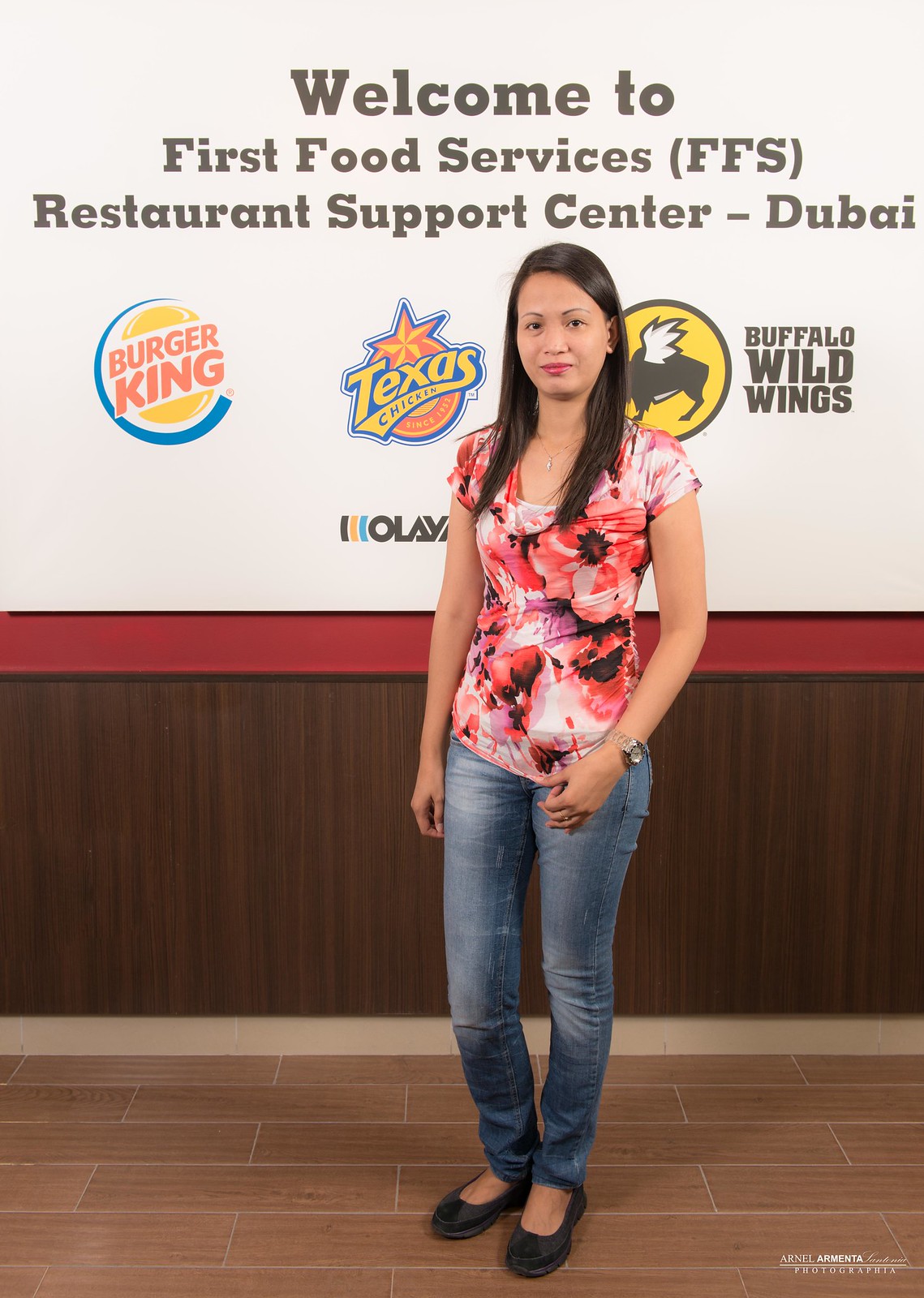The photograph features a young woman standing indoors against a white wall adorned with a poster. She appears to be of Filipino descent, with long black hair cascading just past her shoulders, and she wears a delicate necklace. The woman is dressed in a vibrant floral short-sleeve shirt, predominantly featuring colors like orange, pink, red, and white. She pairs it with faded blue denim jeans and black shoes.

The backdrop behind her features text that reads, “Welcome to First Food Services (FFS) Restaurant Support Centre, Dubai.” Below this header are logos for several well-known fast-food brands. Starting from the left, there is the Burger King logo, followed by the Texas Chicken logo, and then the Buffalo Wild Wings logo. Toward the bottom of the poster, the word "Olay" is visible but partially cut off. The detailed setting and array of logos suggest the photograph was taken in a restaurant support center.